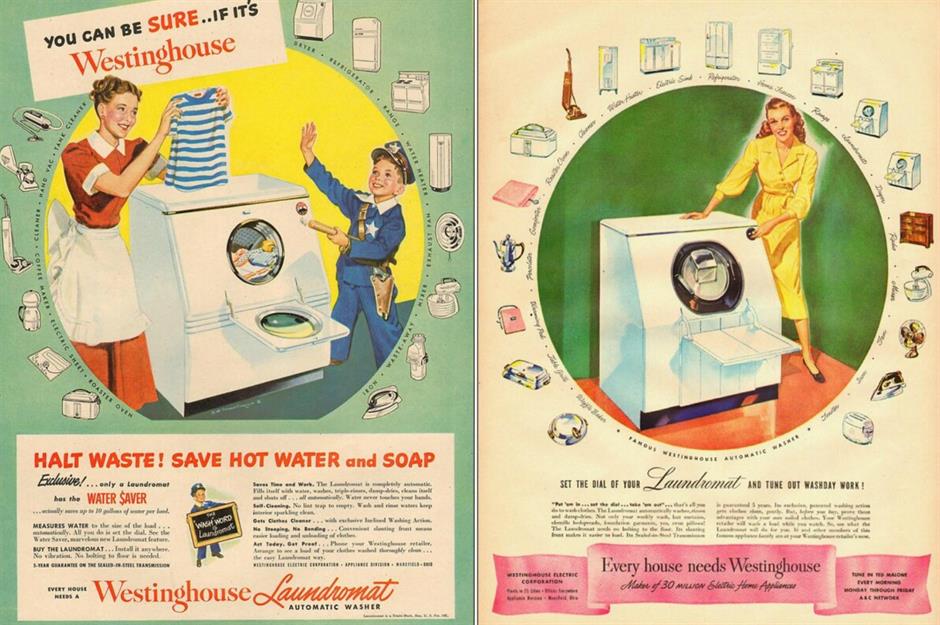This horizontal rectangular frame contains two adjacent full-page Westinghouse Appliance advertisements from the 1950s, showcasing their front-loading washing machines. The left advertisement features a vintage scene set against a green background. At its center, a red-headed woman in a burnt orange dress with a white apron proudly holds up a blue and white striped children's shirt she has just removed from the open washing machine. To her right stands a little boy in a blue police uniform, complete with a white star and blue hat. Above them, a white text box proclaims, "You can be sure if it's Westinghouse." At the bottom, a red text box urges, "Halt Waste, Save Water and Soap," and further text below details the features.

The right advertisement presents another woman, this time in a yellow dress, enthusiastically gesturing towards the same model of front-loading washing machine. The scene is dominated by a circular illustration, similar to the left one. Below, a pink ribbon banner states, "Set, let the laundromat do your work for you," along with smaller text and images of other appliances, emphasizing the ease and efficiency brought by Westinghouse appliances. Both adverts feature a couple of paragraphs of finer print text at the bottom, providing more detailed information about the products and their exclusive water-saving features.